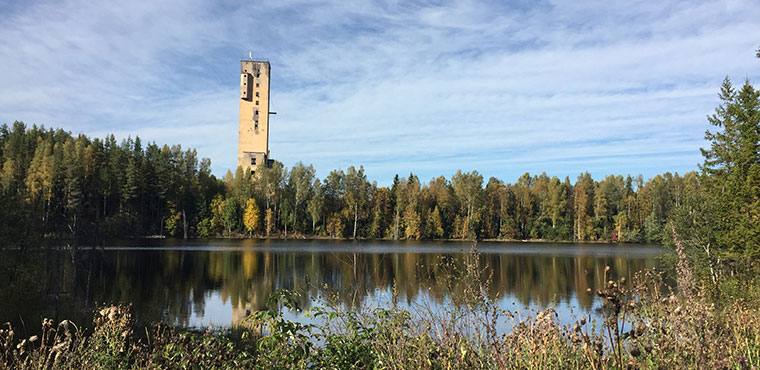The photograph captures a serene, sunlit outdoor scene featuring a large lake at its center. The lake mirrors the lush green tree line and a prominent, aged tan tower that rises from the distant shore. This tower appears dilapidated, with much of its original tan paint chipped away to reveal the gray concrete beneath. Topping the structure is a black railing, and a white flag flutters above it. The foreground of the image includes diverse green vegetation such as water plants, ferns, or tall grasses. On the right side, a healthy pine tree with dense green needles adds to the natural beauty. The sky overhead is a light blue with patches of wispy white clouds. The tower stands out starkly against the forest and sky, suggesting it might be an old lookout or watchtower, possibly once used for military or observational purposes.